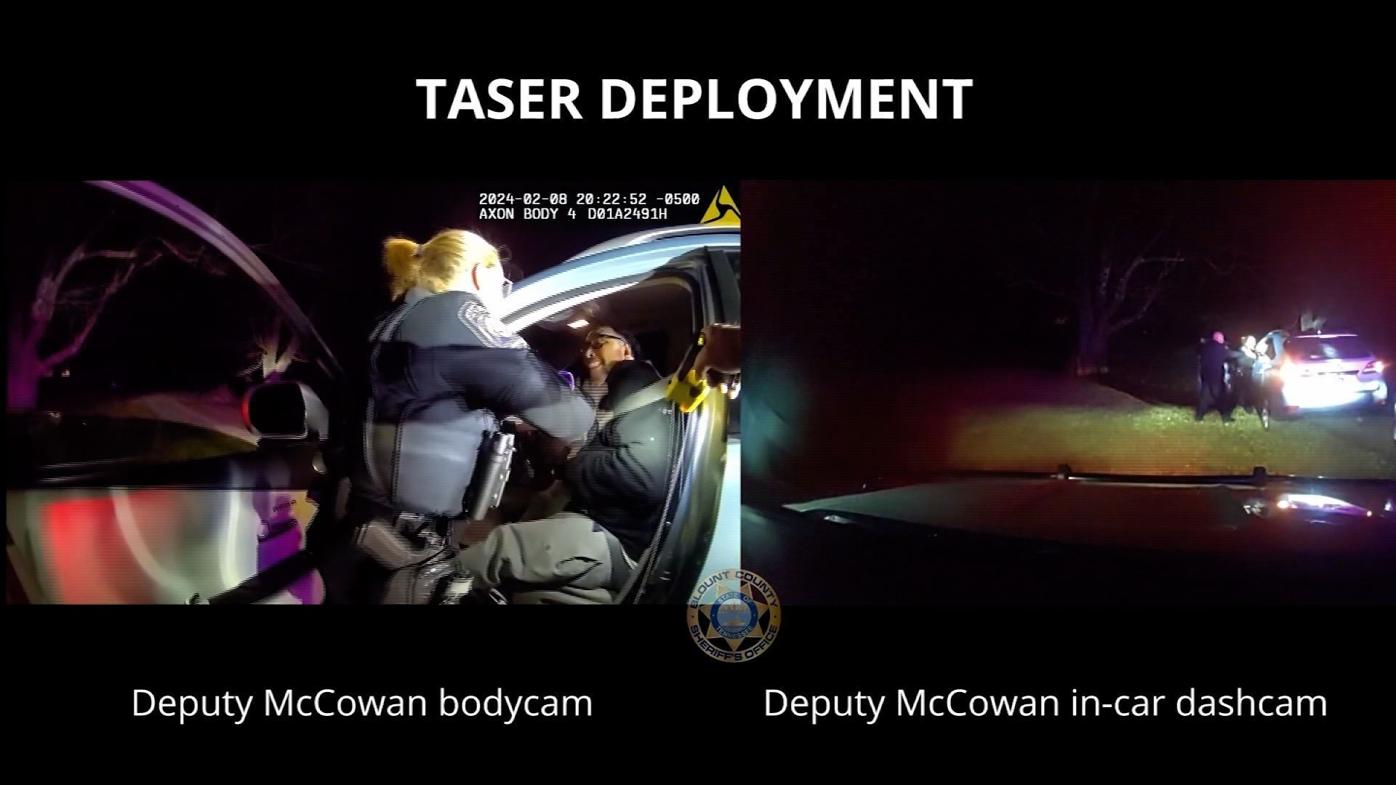The image consists of two still shots against a black background titled "Taser Deployment" with the timestamp "2024-02-08," indicating the event occurred on February 8th, 2024. Both stills are from Deputy McCowan, with the left image labeled "Deputy McCowan Body Cam" and the right "Deputy McCowan In-Car Dash Cam."

The left image, captured from the body cam, shows a close-up of Deputy McCowan, a blonde female officer with a ponytail, wearing tactical gear and glasses. She is engaging with a suspect seated in the driver's seat of a grey vehicle with its door open. The suspect, a man in dark clothing and black-framed glasses, appears uncooperative, prompting Deputy McCowan to use a taser. The setting is dark, suggesting the event occurred at night. 

The right image, from the in-car dash cam, captures the same scene from a wider angle. This view includes the grey vehicle's headlights and taillights, a tree in the background, and some green grass, providing a broader context of the location. Both images juxtapose the close, detailed action from the body cam with the broader, situational overview from the dash cam.